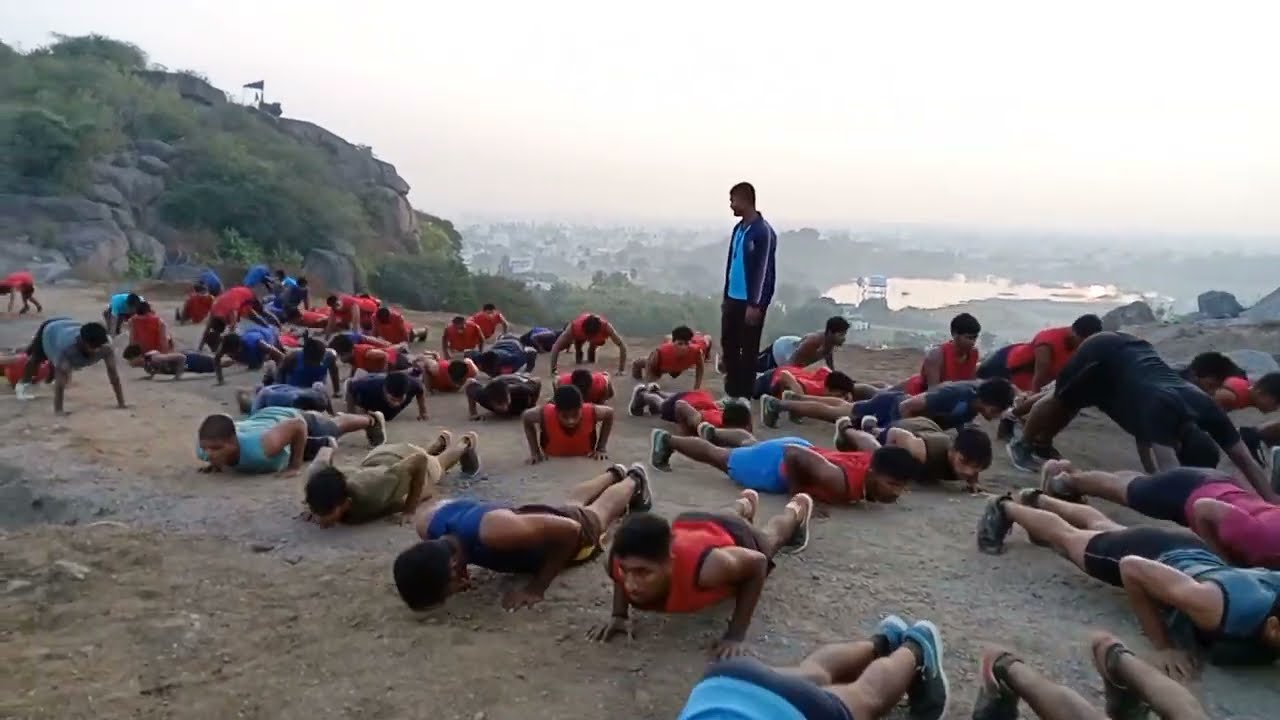In this detailed photograph, a fitness boot camp is underway on a sandy terrain, possibly a sandbar. The foreground is dominated by a large group of people in mid-push-up positions, many decked out in workout attire with sneakers. Most participants are wearing either purple or red shirts, perhaps indicating team colors. The backdrop reveals a city skyline under a hazy sky, with glimmers of sunlight reflecting off a body of water, suggesting early morning or late afternoon. 

To the left, a rocky mountain covered in shrubbery towers with a flag at its summit, adding a rugged landscape element. On the right, a bright yellow sunrise casts a golden hue over the scene, complementing the urban sprawl of rooftops below. Near the center of the foreground stands a man, possibly the instructor, distinguished by his dark blue tracksuit with white stripes, a light blue shirt, and black pants. He wears a whistle around his neck, signifying his leadership role. His watchful gaze over the trainees underscores the disciplined atmosphere of the boot camp session.